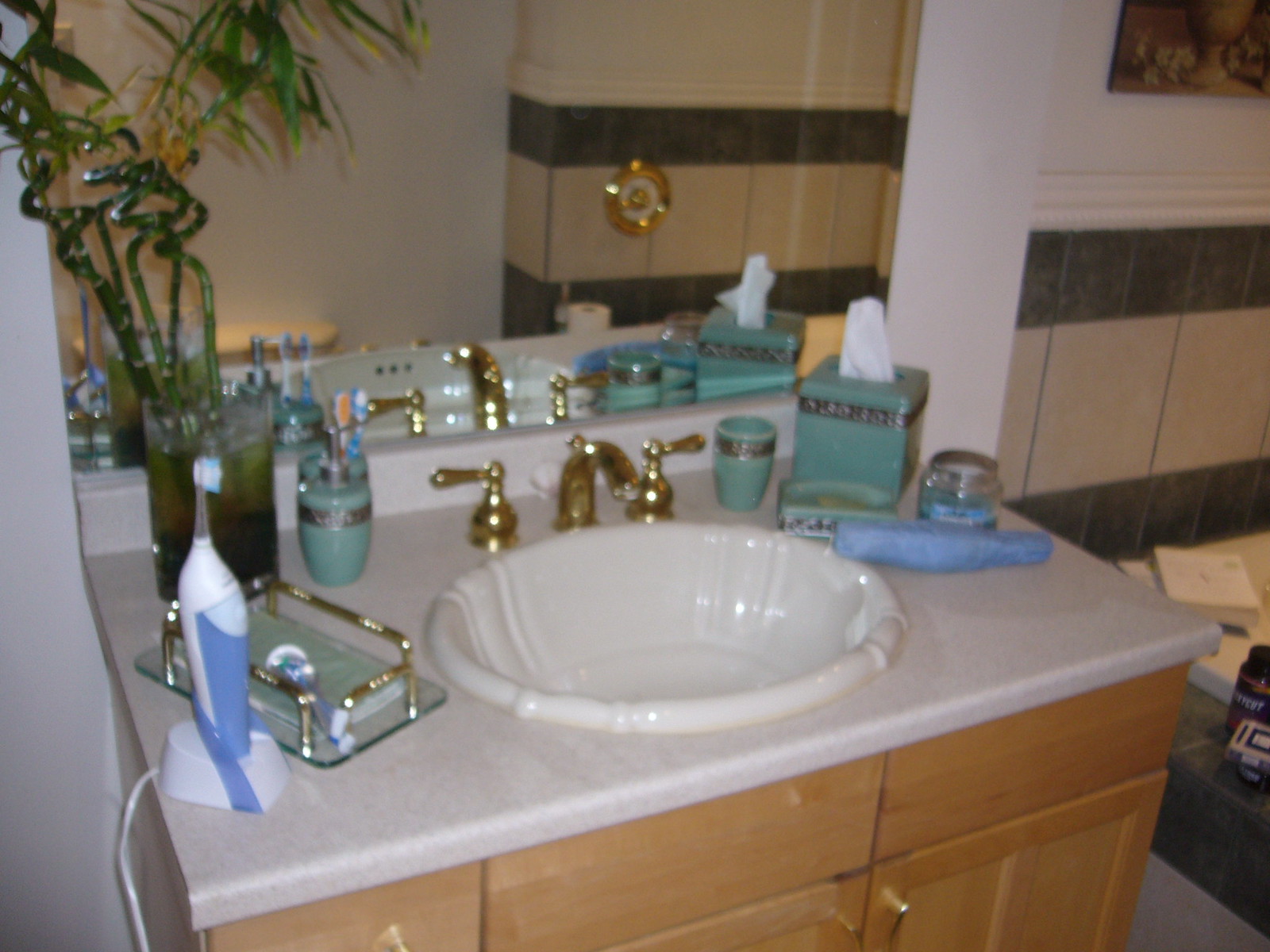This photograph showcases a bathroom that exudes the opulence of an upscale 1980s home. The decor, while characteristic of that era, has evidently been well-maintained, suggesting this could be a modern-day capture. The centerpiece is a white vanity top, subtly marbled with off-white hues, atop which sits an exquisitely ornate circular ceramic sink. This sink is notable for its distinctively thick and decorative lip, likely a rare and luxurious feature.

The gold faucets and vintage-style knobs for hot and cold water add to the overall grandeur, alluding to a bygone era of lavish design. Matching accessories, including a green and silver Kleenex box cover, a cup, a hand soap pump, and possibly a soap tray, contribute to the coordinated aesthetic. A blue candle adds a touch of contemporary charm amidst the vintage elegance.

An electronic toothbrush, notably hefty in design, rests in its holder on the counter, accompanied by spare toothbrush heads. Completing the vignette, the back left corner exhibits a clear glass vase filled with murky water, housing abundant bamboo stalks. This eclectic blend of elements results in a bathroom scene that is both nostalgic and meticulously sophisticated.